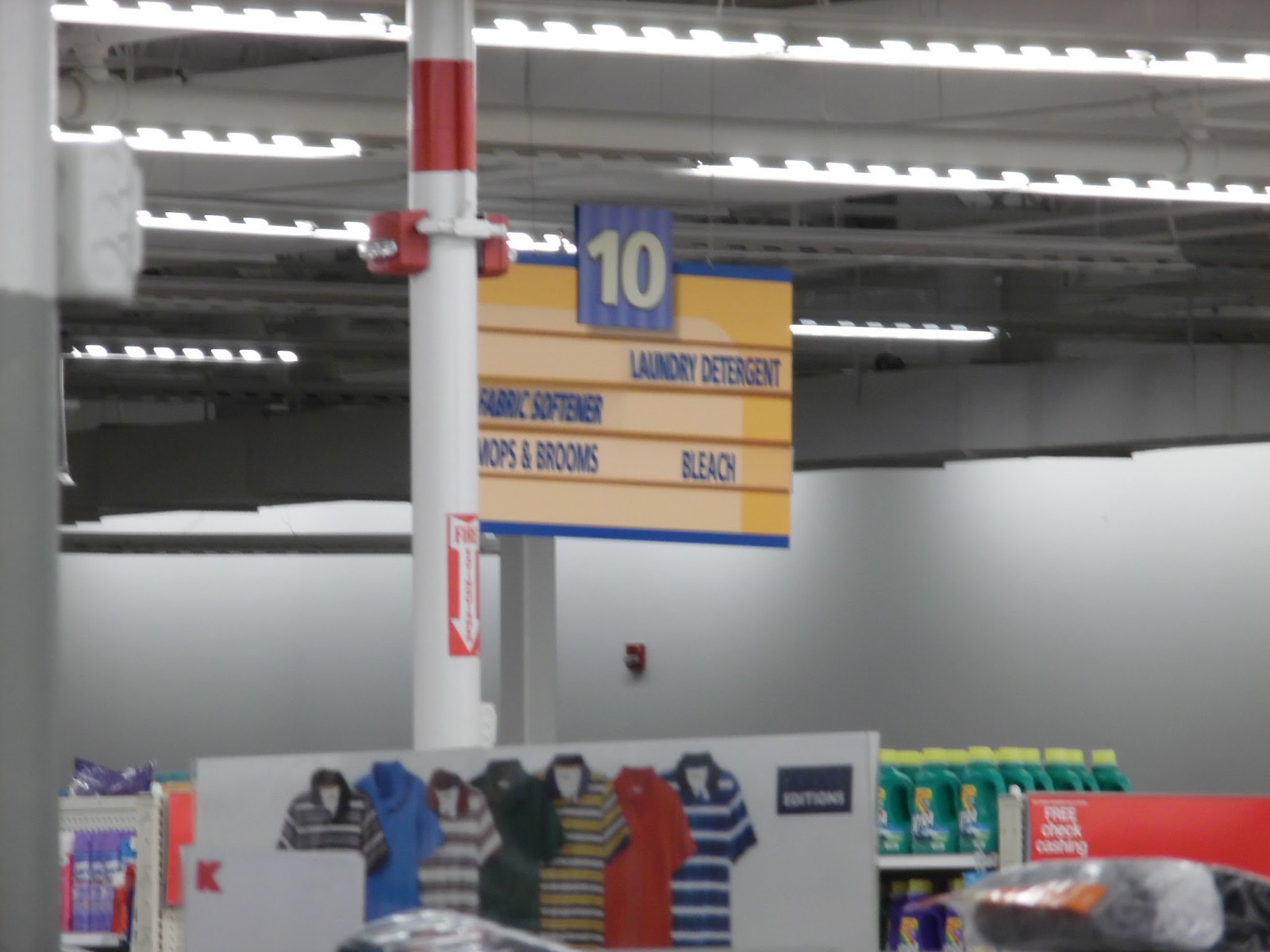The color photograph captures a small segment of a retail store. In the bottom half of the image, there is a display shelf featuring neatly arranged polo shirts. The shirts come in various styles: one has blue and white horizontal stripes, another has light gray and light brown horizontal stripes, while others are solid colors including red, black, and blue. On the right side of the photograph, another shelf displays what appears to be a green bottle of Gain brand laundry detergent. To the left, a tall white pole stands with a sign attached, indicating Aisle 10. The sign lists the store items found in this aisle: laundry detergent, bleach, fabric softener, mops, and brooms.